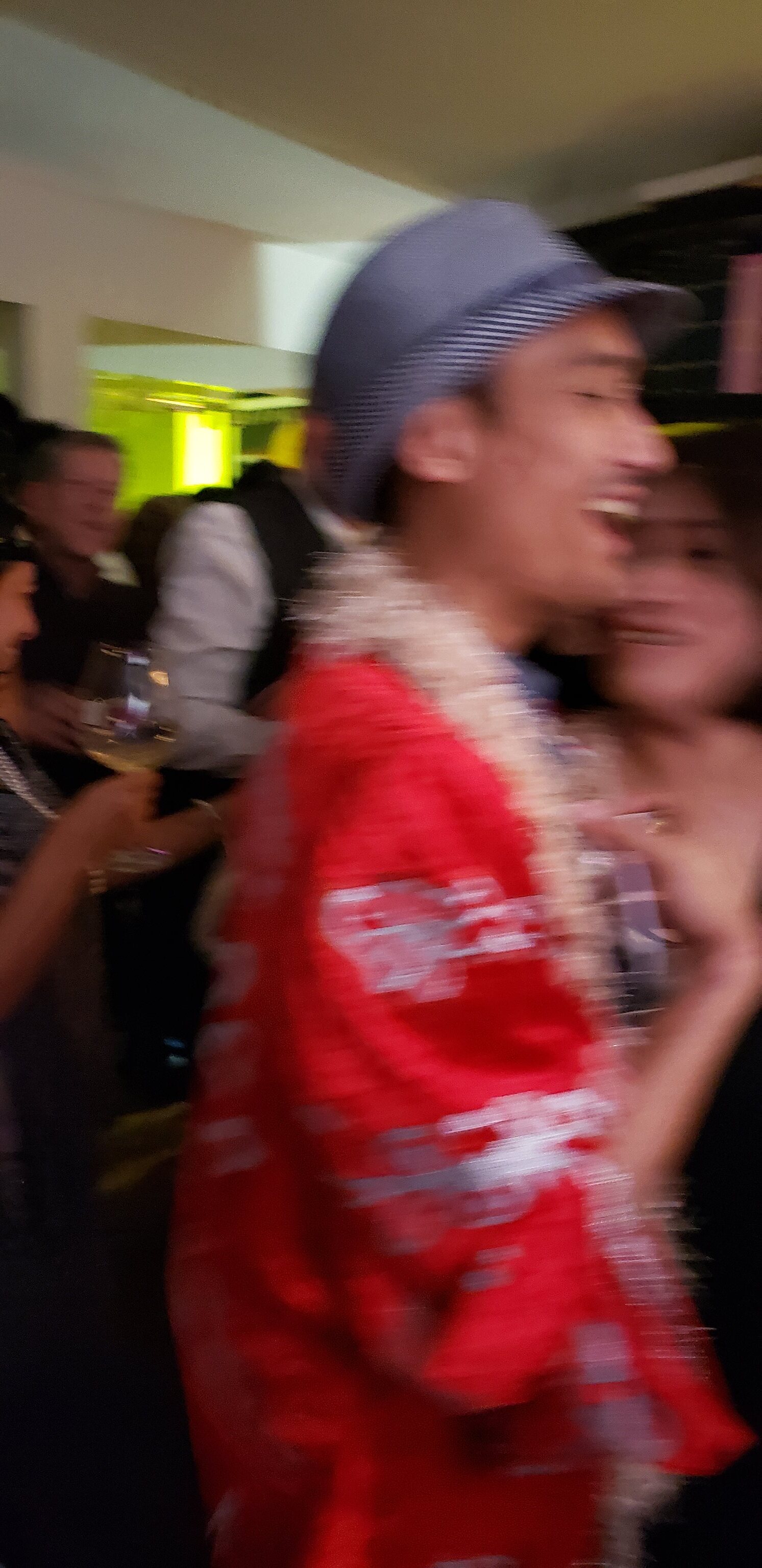This color photograph, though blurred, captures a lively moment in an indoor setting. The central focus is on the left side of a man, whose indistinct features convey a sense of movement and energy. He wears a grey and white rimmed hat paired with a red garment that resembles either a football shirt or a tunic, adorned with silvery logos. Draped around his neck is a decorative garland, possibly petalled, adding a festive touch to his attire.

Just below him, the partial view of a woman’s head with short, dark hair, and a glimpse of her neck, is visible. In the background to the right, several indistinct figures can be seen, contributing to the bustling atmosphere. The scene is underscored by a brown and white roof and a yellow-green light that adds warmth to the setting. The photograph hints at an event where people have gathered, likely a pub, restaurant, or party, capturing the joyful, communal spirit of the occasion.